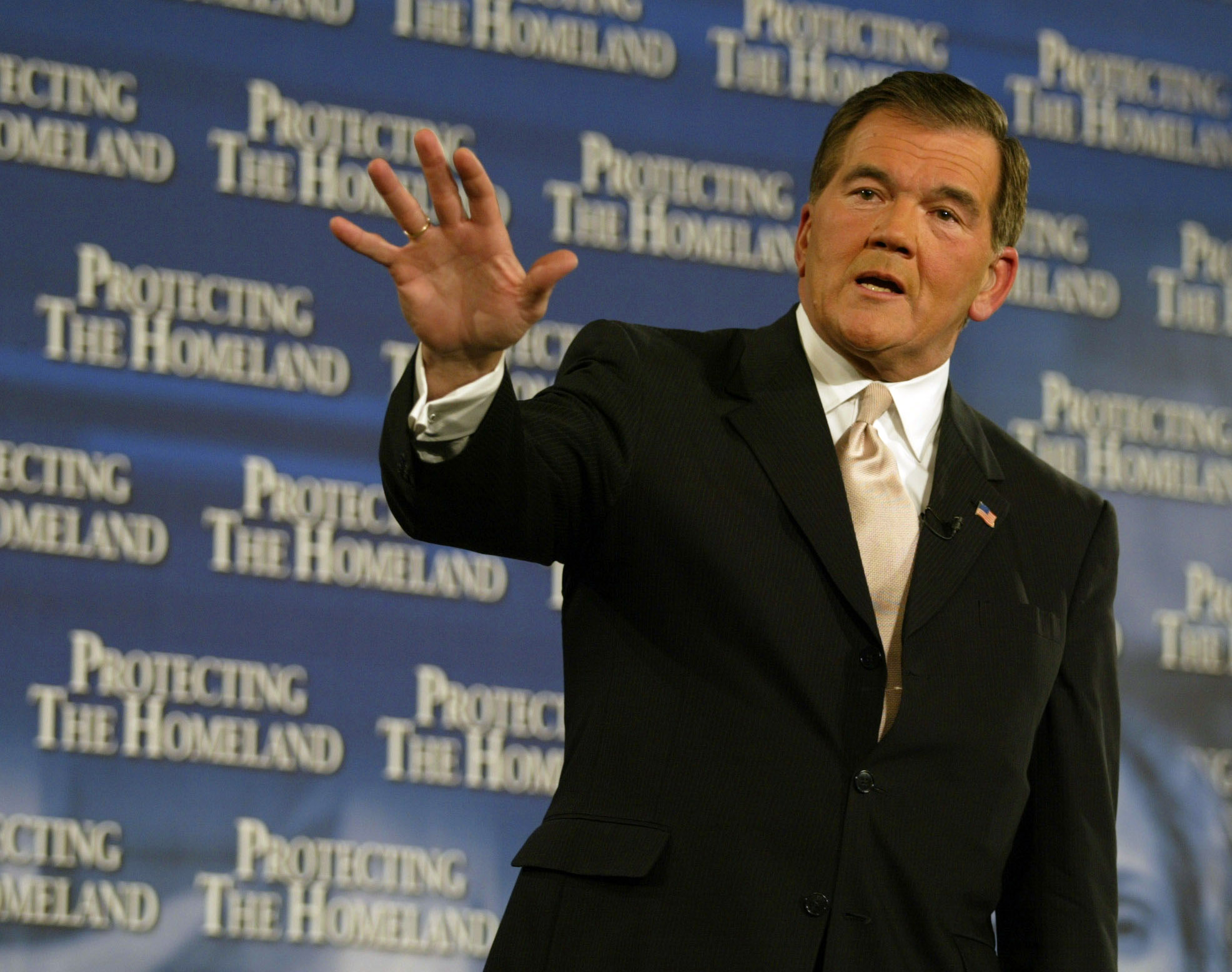The photograph depicts an older Caucasian man, possibly in his 60s, standing in front of a blue banner inscribed with the phrase "PROTECTING THE HOMELAND" in white serif font, repeated multiple times. The man, who has short grayish-brown hair and bushy gray eyebrows, is dressed in a black suit jacket with a white collared dress shirt underneath. He is wearing a gold-colored tie and has an American flag pin on the right lapel of his suit jacket. His left hand is raised, palm out, and he appears to be in the middle of speaking, with his mouth slightly open. A small black microphone is visible on his left chest. The overall impression is that he might be a politician addressing an audience.